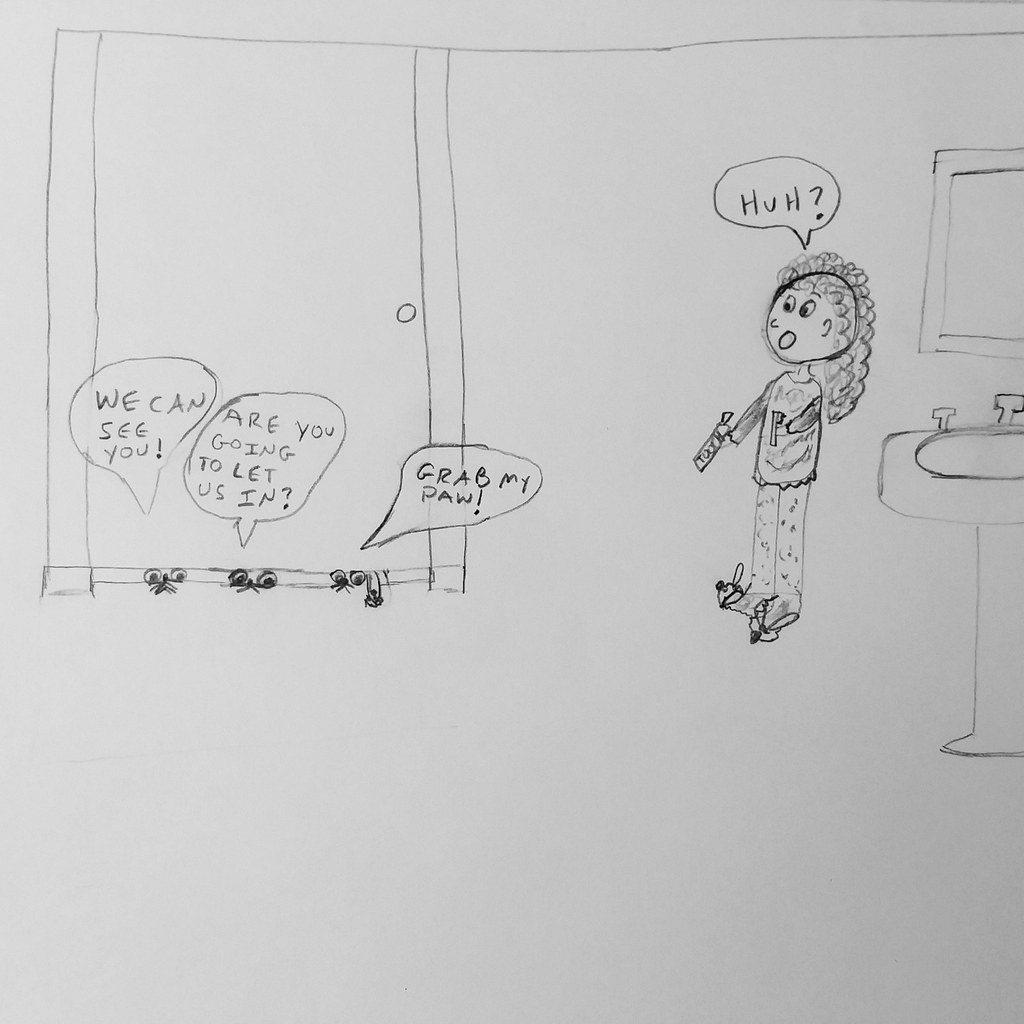This large, borderless square image features a black and white hand-drawn cartoon, possibly created with pencil or pen. On the left side, there's a simplistic drawing of a door, indicated by a small circular doorknob and vertical lines, while under the door, three sets of critter eyes with paws sticking out are visible. Each set of eyes has a speech bubble, with the left one saying "We can see you!", the middle one asking "Are you going to let us in?", and the right one exclaiming "Grab my paw!" To the right of this scene, a surprised woman with swirly long hair stands in pajamas and bunny slippers, holding a toothbrush and toothpaste. She has a speech bubble that simply says "Huh?" and wide-eyed expression. To her far right, an outline of a bathroom sink with a mirror is also depicted, completing the bathroom setting where the comic interaction is taking place.